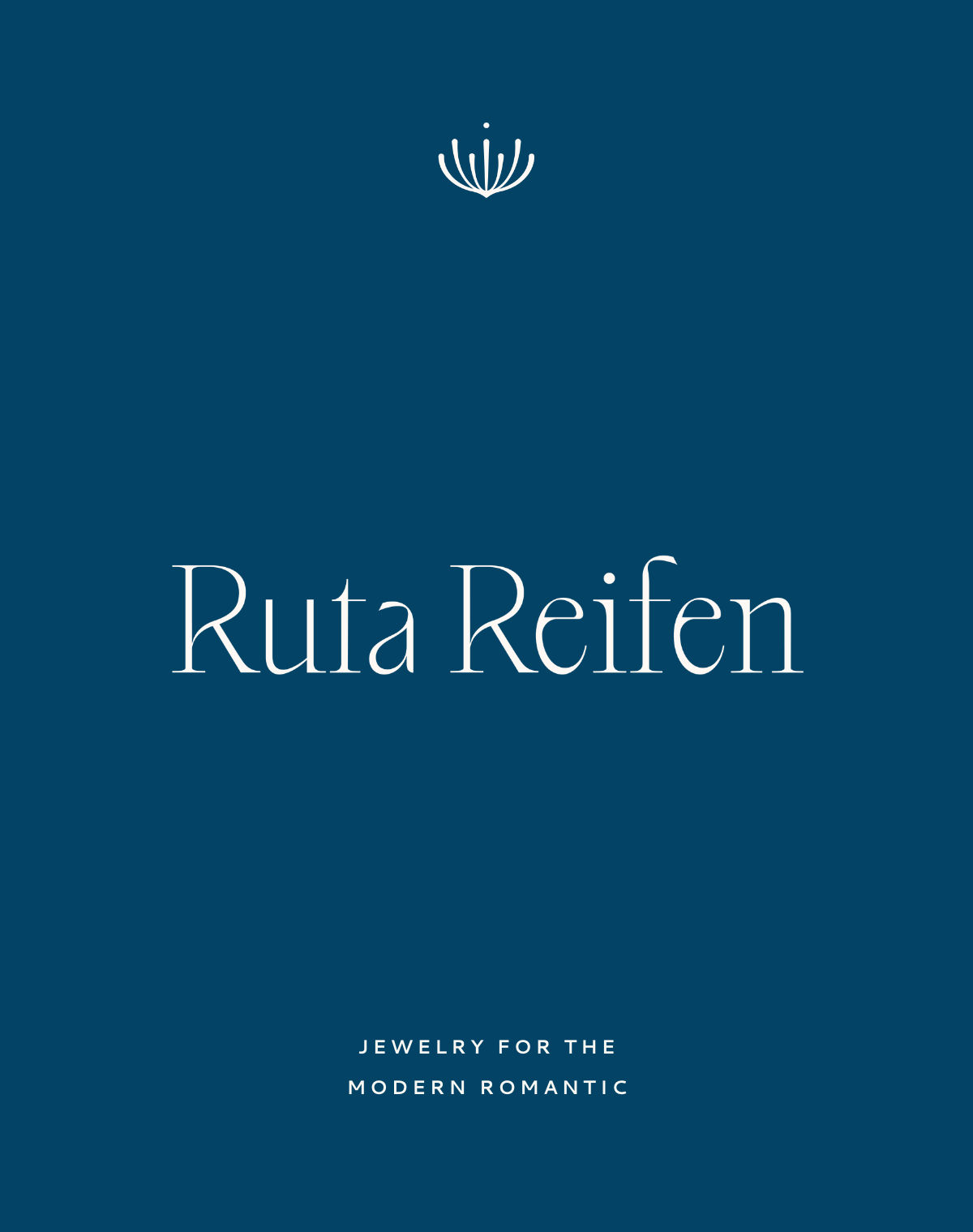This image features a minimalist advertisement for a jewelry brand set against a solid medium navy blue background with subtle teal undertones. Dominating the top portion is a distinctive white U-shaped symbol with vertically extending, variously curved projections, resembling a stylized or abstract floral petal design. Centered prominently in elegant white serif font are the words "Ruta Reifen," with both 'R's capitalized. Below, near the bottom and also centered, is the tagline "Jewelry For The Modern Romantic," rendered in a much smaller, all-capitals sans-serif font. This stylish display likely serves as a cover or promotional material, capturing a sleek and sophisticated brand aesthetic.